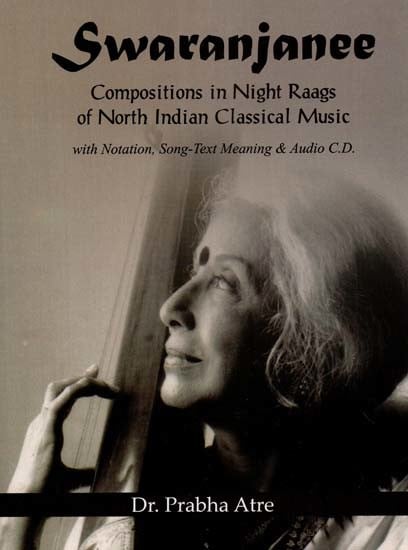The image is a black and white cover of a book titled "Swaranjanee," spelled S-W-A-R-A-N-J-A-N-E-E, displayed in black text at the top. Beneath the title, it reads, "Compositions in Night Raags of North Indian classical music with notation, song text meaning, and audio CD." At the bottom, within a thick black line, the name Dr. Prabha Atre is prominently displayed. The cover features a photograph of an older woman with white hair, bearing a distinctive Hindu mark on her forehead. She is in profile, facing the left, her gaze directed slightly upwards as if looking out a window. She is poised and composed, holding and fingering the strings of a traditional instrument with her right hand, possibly in a teaching or demonstrative manner, adding to her centered and authoritative presence in the image.